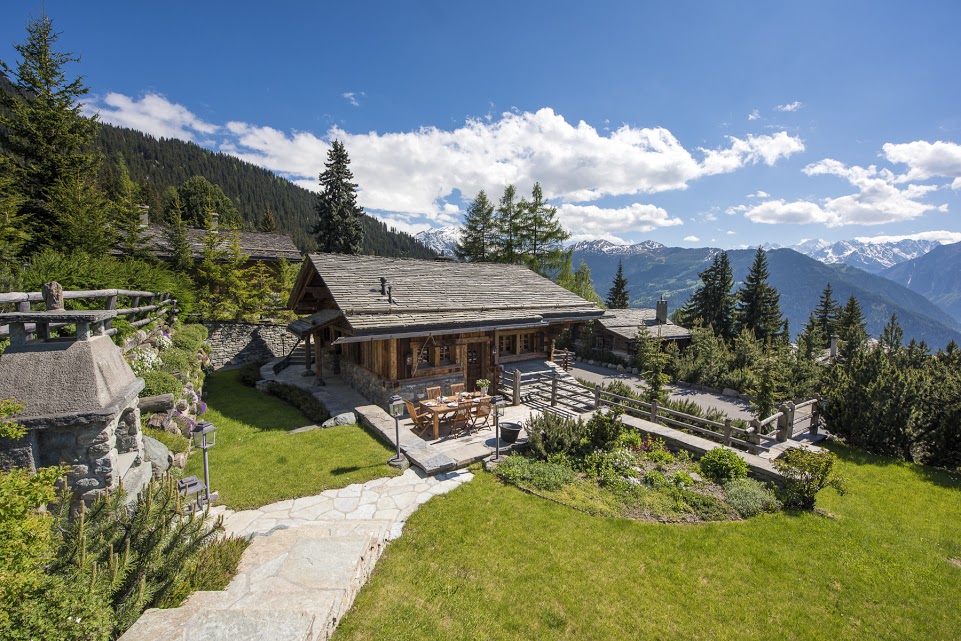This captivating photograph showcases a picturesque wooden cabin nestled in a lush, green landscape and surrounded by towering pine trees, with majestic, white-tipped mountains looming in the background under a bright blue sky scattered with fluffy white clouds. The log house, perched on a hill, boasts polished brown beams and a darker greyish wooden roof, exuding rustic charm. The front of the cabin features an inviting wooden deck, complete with a table surrounded by several chairs, thoughtfully set for a meal. A neatly maintained green lawn spreads out in front, bordered by vibrant green plants and more pine trees of varying heights. A stone pathway meanders up to the cabin, enhancing the idyllic beauty of the scene. Off to the side, there is a smaller structure, partially obscured, and in the middle ground, another cabin is visible, adding to the sense of a serene, mountain retreat. The overall ambiance is one of tranquility and natural beauty, accentuated by the clear, sunny day.